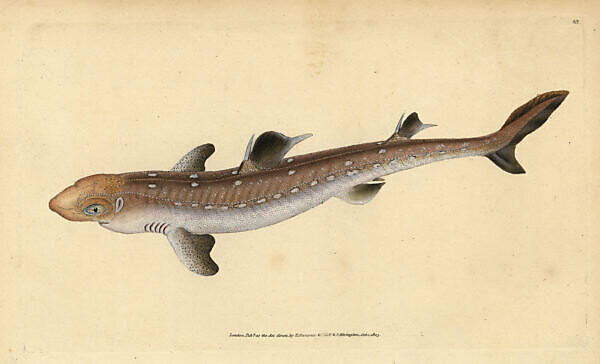This image depicts a detailed sketch of a fish, possibly a shark, viewed from a side angle with a slightly top-down perspective. The fish is swimming from left to right, with its head on the left and its tail on the right. The fish has a large head with a lighter brown color while the rest of its body is grey, marked with various white spots. It has a prominent dorsal fin, gills, and an eye visible on the side. Additional fins are positioned just behind the gills on both the upper left and right sides, along with two fins on the top, one fin below, and a bifurcated tail with two fins. The background of the image is a worn, tan or cream-colored paper. At the bottom of the picture, there is a grey teardrop shape containing an 'M' and tiny black letters that are too small to read. There also appears to be a possible number in the upper right corner, which is also too faint to decipher.